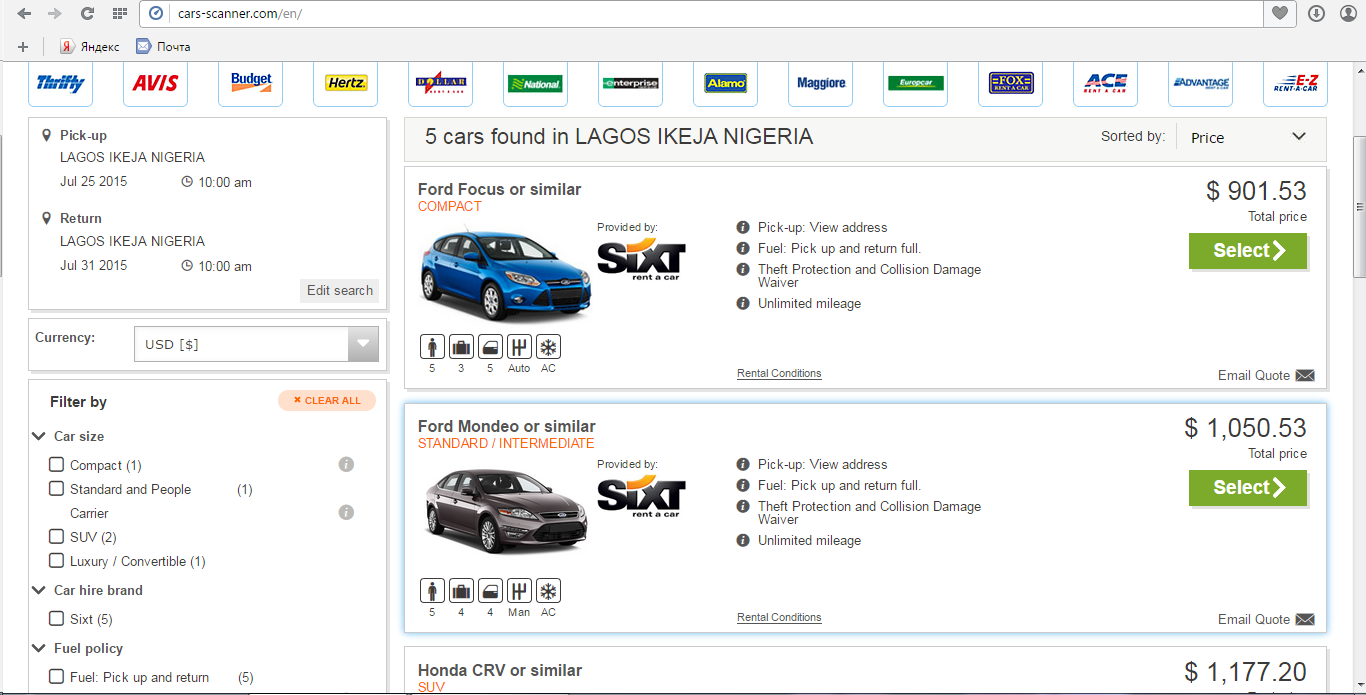This screenshot captures a comprehensive car rental comparison website at the URL car-scanner.com. At the top of the webpage, a white URL bar is clearly visible, signifying that the site is fully loaded and ready for user interaction. The header prominently displays a diverse array of over a dozen recognizable car rental logos, including Thrifty, Avis, Budget, Hertz, Dollar, National, Enterprise, Alamo, Magura, Green One, Fox Rent-A-Car, East Rent-A-Car, Advantage, and Easy Rent-A-Car, illustrating the wide range of options available.

On the left side of the webpage, there's a section dedicated to selecting pick-up and return details, accompanied by an 'Edit Search' button for revising search criteria. Immediately below this, the layout is divided into two primary columns, with the left being the larger of the two. At the end of this section, there's a currency drop-down button enabling users to select their desired currency.

The filter section is designed for detailed customization, allowing users to refine their search using multiple criteria. Users can filter by car size, car rental brand, and fuel policy, each presenting as intuitive drop-down menus and checkboxes. The car size options include 'Compact,' 'Standard,' 'SUV,' and 'Luxury,' while the car rental brand category features a checkbox for '6T'. The fuel policy options provide checkboxes for 'Fuel pick-up' and 'Fuel return,' empowering users to choose based on their preferred fuel arrangements.

In summary, this image captures a user-friendly car rental comparison tool brimming with various filter options and broad rental choices, presented in an organized and accessible manner.